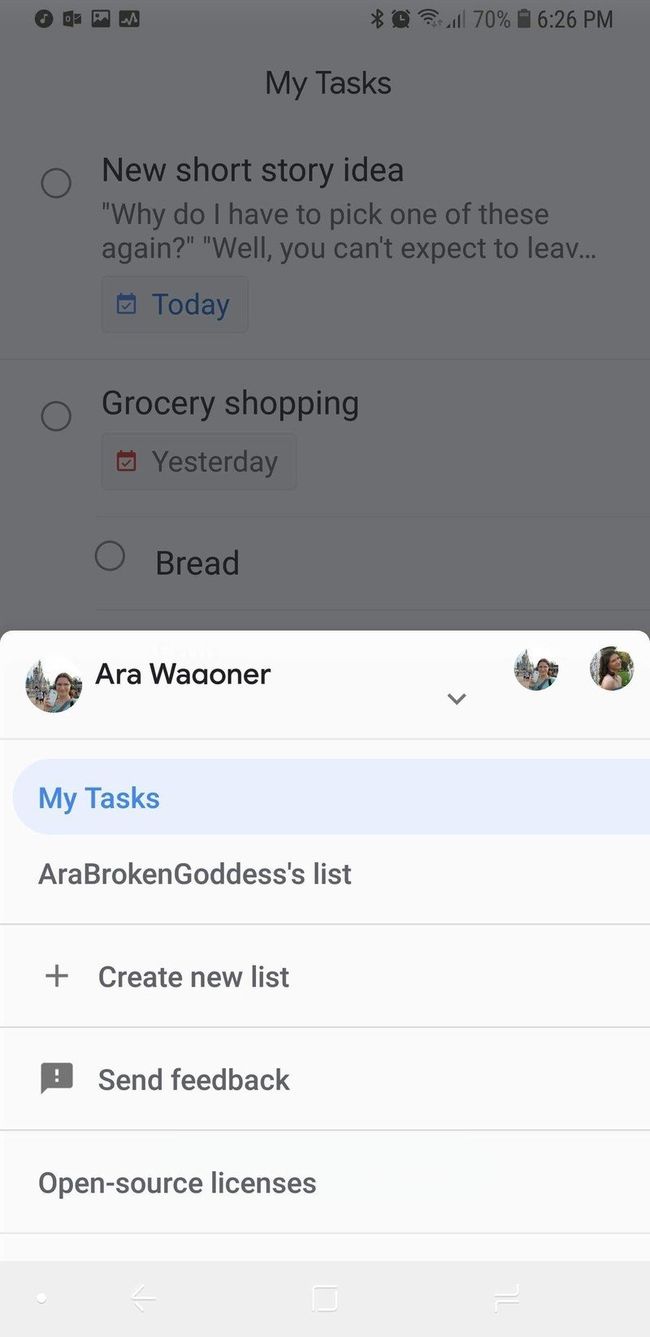The image depicts a smartphone screen with a white background. At the top of the screen, several status icons are visible, including a music icon, an Outlook icon, a screenshot icon, a Bluetooth icon, an alarm icon, a Wi-Fi icon, a network signal indicator, and a battery percentage display showing 70%. The current time is 6:26 PM.

The main application displayed is a task management app titled "My Task." The app's interface shows various task options in black text. The first task listed is "New Short Story Idea," followed by a somewhat incomplete thought: "Why do I have to pick up one of these again well you can't expect to live." Below this, a blue button labeled "Today" is visible. The second task option says "Cross out shopping," and beneath it is another button labeled "Yesterday." There is also a checklist item called "Bread."

In the foreground, occupying the bottom half of the image, is a smaller overlay page. This page features a profile picture of a person named Ara Wa Yona on the left, with an icon representing another person on the right. The text on this page includes options such as "My Task," "Ara Brokens Goldest List," "Create New List," "Send Feedback," and "Open Source Licenses." These options are written in grey, except for "My Task," which is highlighted in blue.

Overall, the image provides a detailed view of the task management app's interface, along with a snapshot of the smartphone's status indicators.